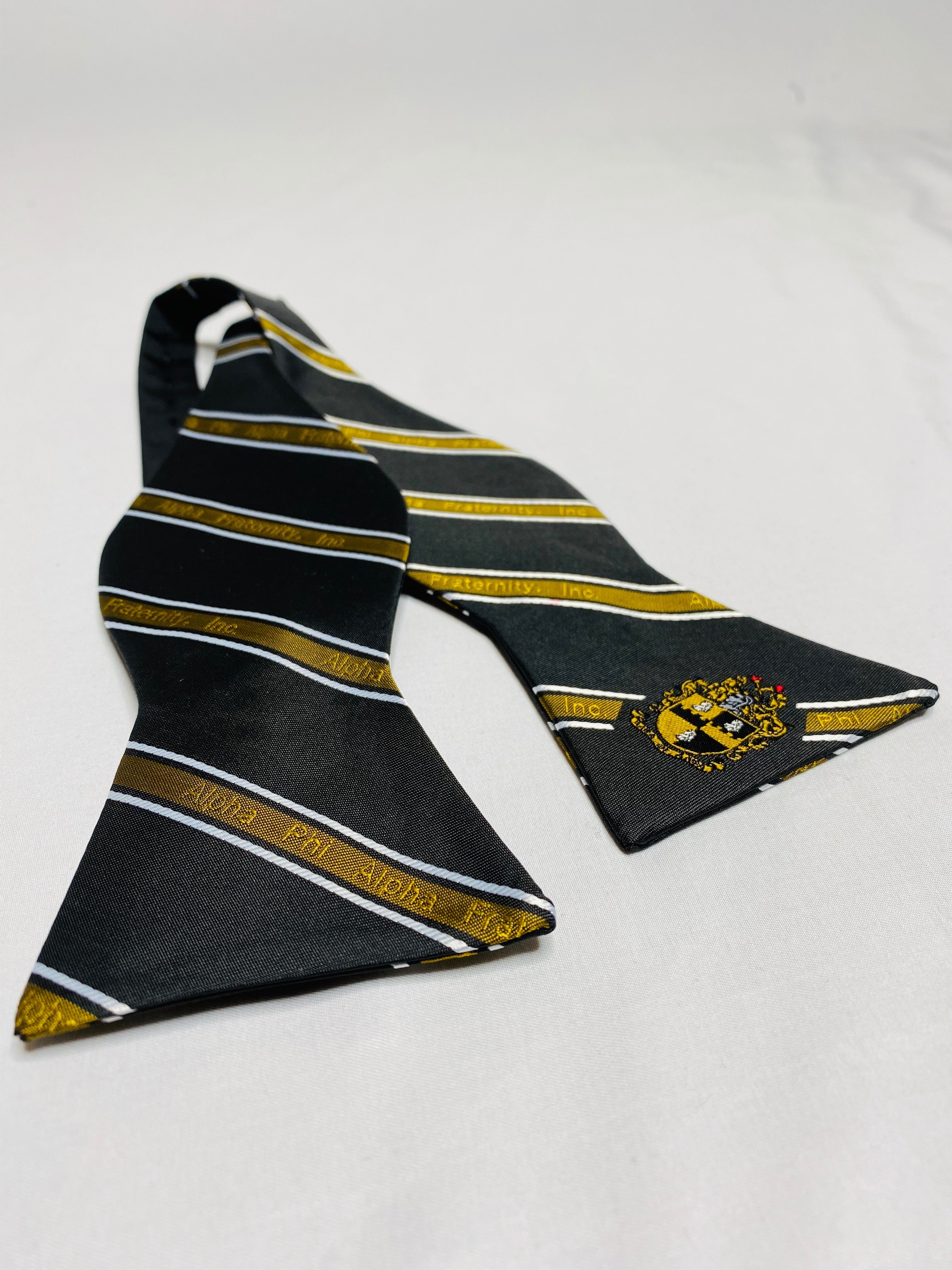The image features a black bow tie laid out on a white surface, possibly a sheet or linen, with faint wrinkles adding texture to the background. The bow tie is untied, displaying its two ends and a rounded central knot. The fabric is shiny, predominantly black, adorned with diagonal yellow stripes edged with white trim. These stripes repeat the text "Alpha Phi" in an alternating pattern. On the right end of the bow tie, there is a black and yellow crest resembling a badge or shield, featuring design elements such as knight helmets. The overall look suggests association with a fraternity, giving the tie a formal and emblematic appearance.